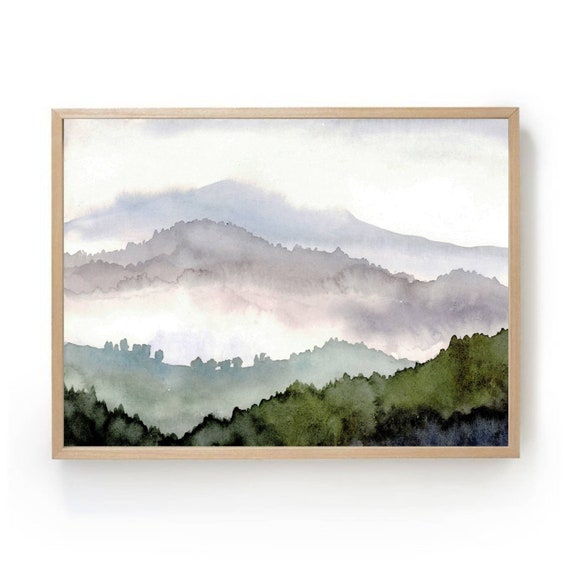This is a detailed photograph of a landscape watercolor painting framed in a light wood, possibly birch, frame. The painting portrays a series of receding mountain ranges and cloud formations layered and fading into the background. The closest foreground features a densely vegetated hill with rich dark green and blue hues, representing treetops and forest greenery. Moving further back, a secondary ridge appears in a hazy, grayish-green, with visible tree silhouettes along its crest. Beyond that, the scene softens into a misty landscape where pale purple and light foggy whites blend into another blurred and distant mountain range. At the backdrop, faint purplish mountains emerge, partially obscured by a cloudy sky, where the clouds appear white below and darker above, mimicking the peaks and valleys of the earth beneath. The painting exudes a minimalist yet evocative atmosphere, skillfully capturing the gradient of colors and the ethereal transition from the dense vegetation to misty mountains and sky.